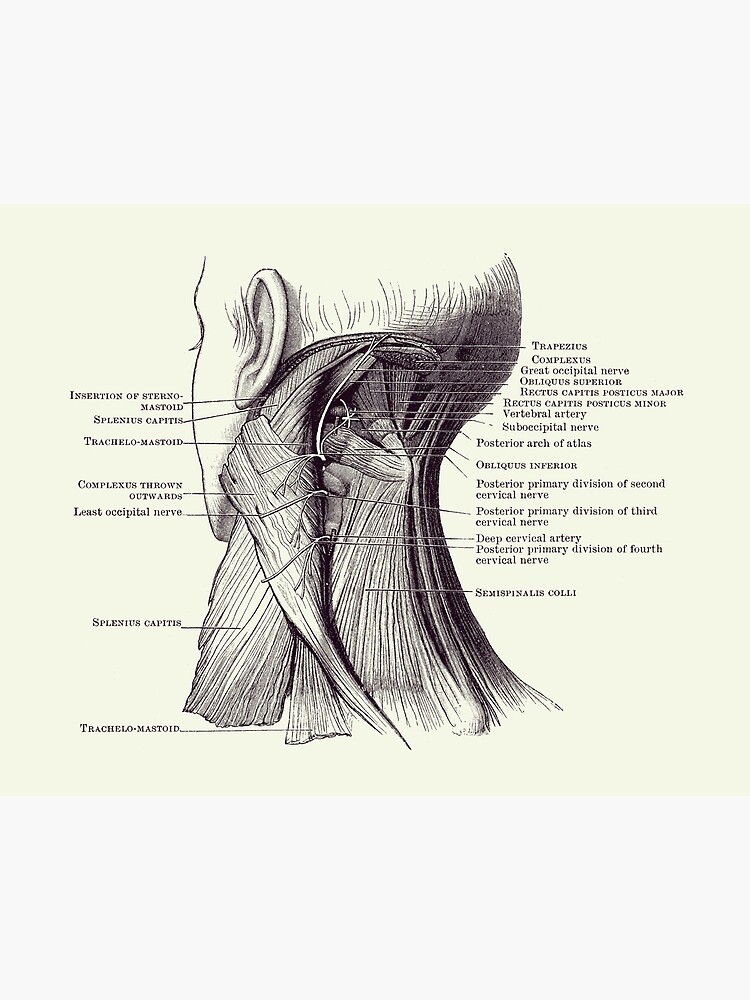This detailed anatomy illustration showcases the lower part of the human head and neck, viewed from the back. Drawn in a simple pen or pencil style on cream-colored paper, the diagram meticulously displays the layers of skin, muscles, tendons, and nerves. The image peels back these layers to reveal intricate structures such as the trapezius, complexus, great occipital nerve, and oblique superior nerve, all clearly labeled with detailed descriptions. The illustration is reminiscent of those found in medical textbooks and aims to provide an in-depth understanding of the anatomical components of the neck. Despite some blurred text, the diagram remains a comprehensive visual guide to these complex systems.